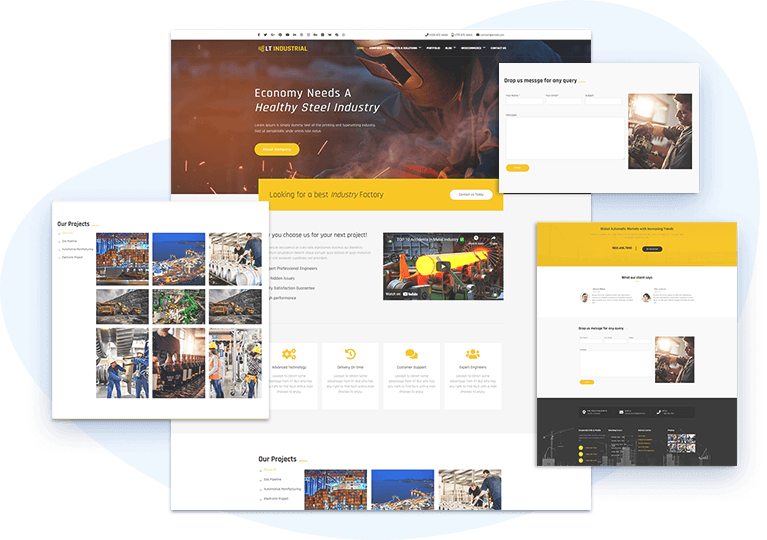The image depicts a multi-page website belonging to LT Industrial. The top section of the first page displays the company's name prominently. The background features a vivid image of a welder wearing a welding helmet, with bright sparks flying around him. Overlaid text emphasizes the significance of a robust steel industry for a healthy economy. Below this is an orange bar, though its text is unreadable. The section beneath the bar includes the phrase "Looking for the best industry factory," accompanied by an image of a factory.

The second page is more text-centric, featuring the statement "Choose us for your next project," with boxes underneath that showcase gold icons and accompanying text. 

Following that is a page dedicated to their projects, with actual photographs of their factory and employees engaged in steelwork. Additionally, another page features a layout with gold at the top, white in the middle, and black at the bottom, where a prominent image of a man working stands out. The top of this section also repeats the same image.

There is a call to action mentioning something about messaging for queries, although the exact wording is unclear. Finally, the bottom section of the site presents a large, colorful photograph labeled "Our Projects," displaying real-life examples of their work.